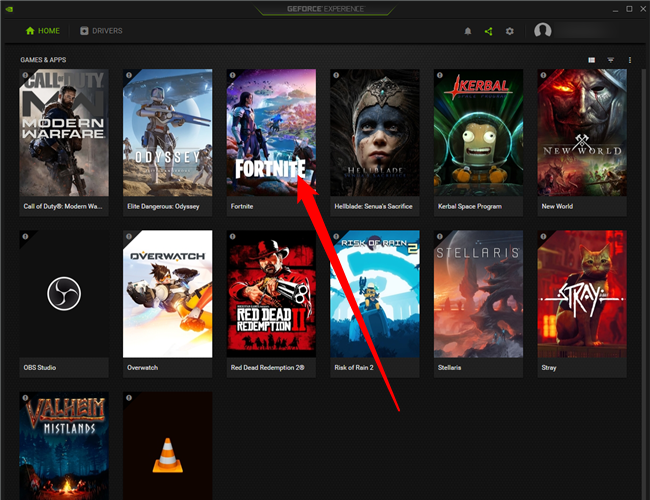**Caption:**

This image is a detailed screenshot of what appears to be a gaming website's interface. The website has a sleek, black background. At the top of the interface, there is a navigation bar with several icons and options. On the left, a home icon is labeled "Home," followed by another labeled "Devices." On the top-right corner, the user interface includes a circular profile picture, a search bar, a settings gear icon, a notifications bell, and a menu icon consisting of three dots in a triangular formation.

Below the navigation bar, there are three rows showcasing cover images for various games. The top row begins with a section titled "Games and Apps." Prominently featured is the cover for "Call of Duty: Modern Warfare," followed by "Odyssey" and "Fortnite." Notably, the "Fortnite" cover has a large red arrow superimposed on it, with the arrow pointing downwards to the bottom of the image. Next in the row are the covers for "Hellblade" and "Kerbal Space Program."

The second row includes covers for "New World," "CBS Studio," "Overwatch," "Red Dead Redemption 2," "Risk of Rain 2," "Stellaris," and "Stray." The third and final row includes "Valheim Mistlands" and ends with an icon of a red, white, and orange traffic cone.